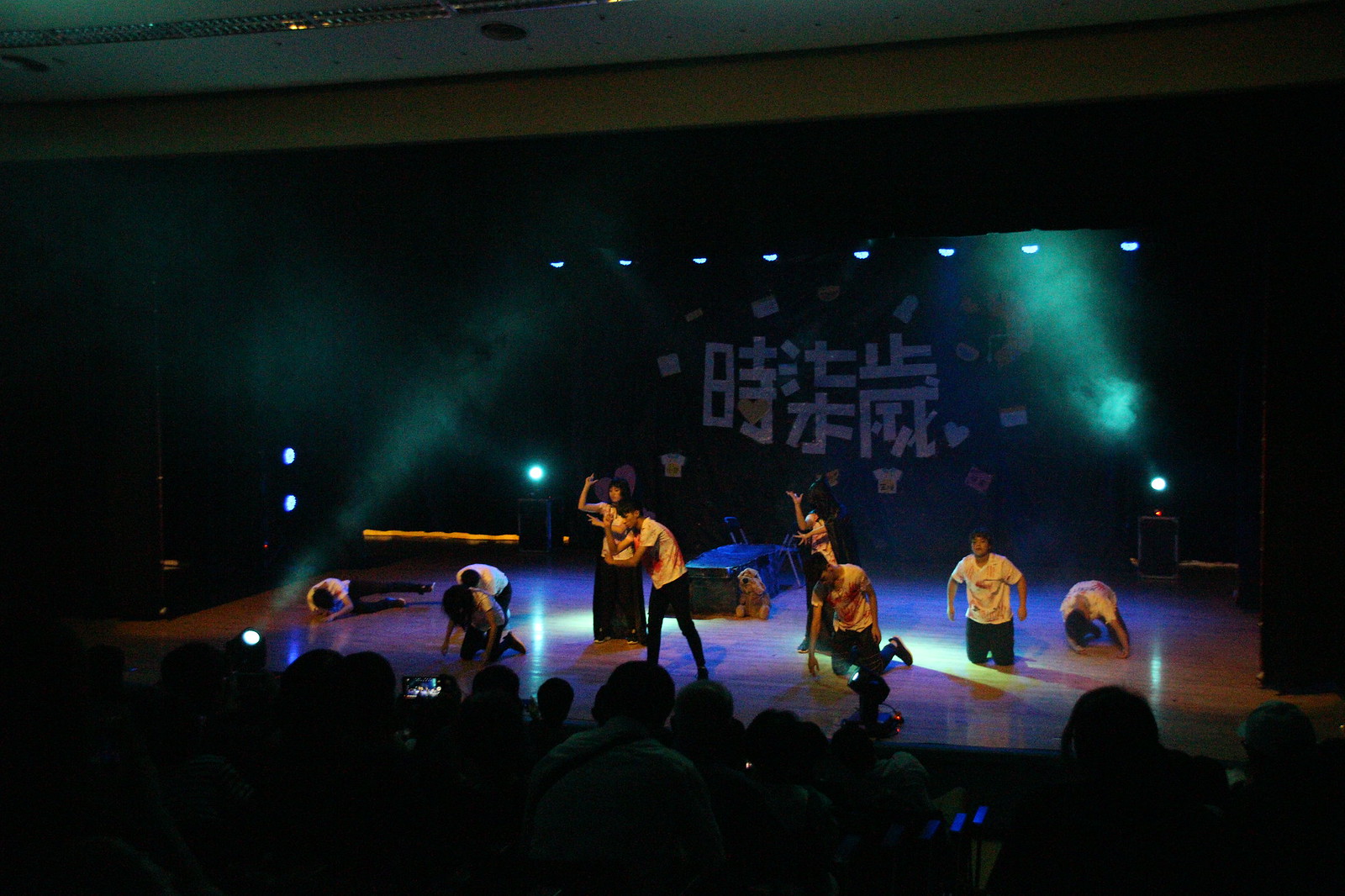The image showcases an indoor stage performance set in Asia, characterized by Chinese or Japanese lettering prominently displayed in white across a dark backdrop. A series of spotlights, including green ones, illuminate the stage, casting multicolored hues such as blue and yellow onto the wooden floor. Approximately nine performers are captured in various dynamic poses, engaging in what appears to be a dance or play without instruments. Notably, a woman in a yellow shirt and black pants stands in the center with her arms lifted, while others—also in yellow shirts and black pants—kneel or crouch, hands on the floor or making intricate motions. Some performers are standing, adding to the visual diversity of the scene. In the foreground, silhouetted heads of seated audience members are visible, enhancing the sense of a live, immersive performance. The stage is also adorned with a trunk, a stuffed animal, and chairs, adding to the theatrical setting.